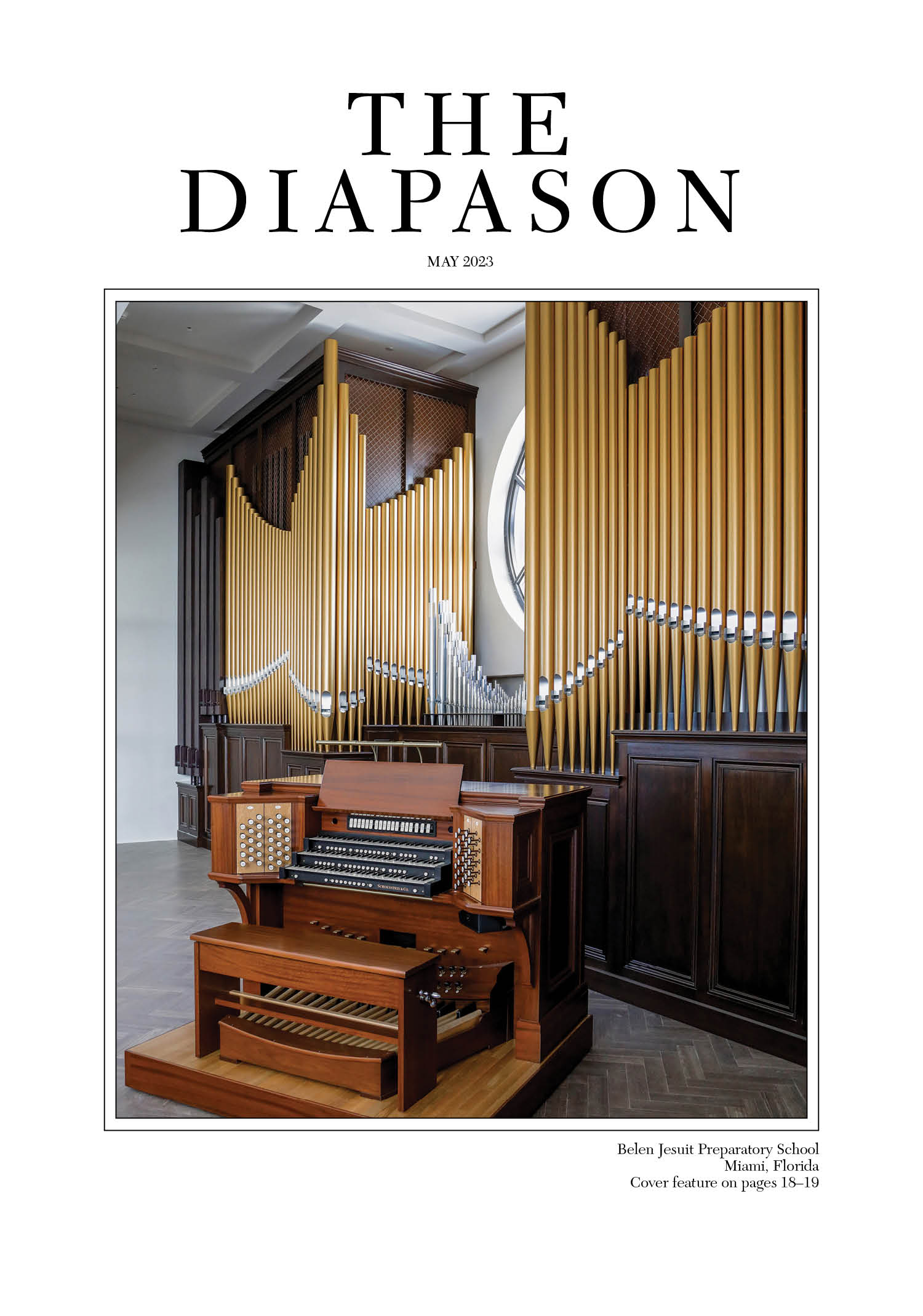The magazine cover prominently features a large photo of an impressive church organ with numerous gold pipes arranged vertically. The organ’s cabinetry is a dark brown wood, housing three keyboards, various knobs, and buttons. Positioned in the lower left is a smaller, medium brown wooden keyboard with a matching bench on a brown floor. The image also reveals a window behind the organ pipes. Across the top of the cover, bold black text reads "The Diapason," with smaller text underneath indicating "May 2023." In the lower right corner, additional black text notes, "Belen Jesuit Preparatory School, Miami, Florida. Cover feature on pages 18-19."